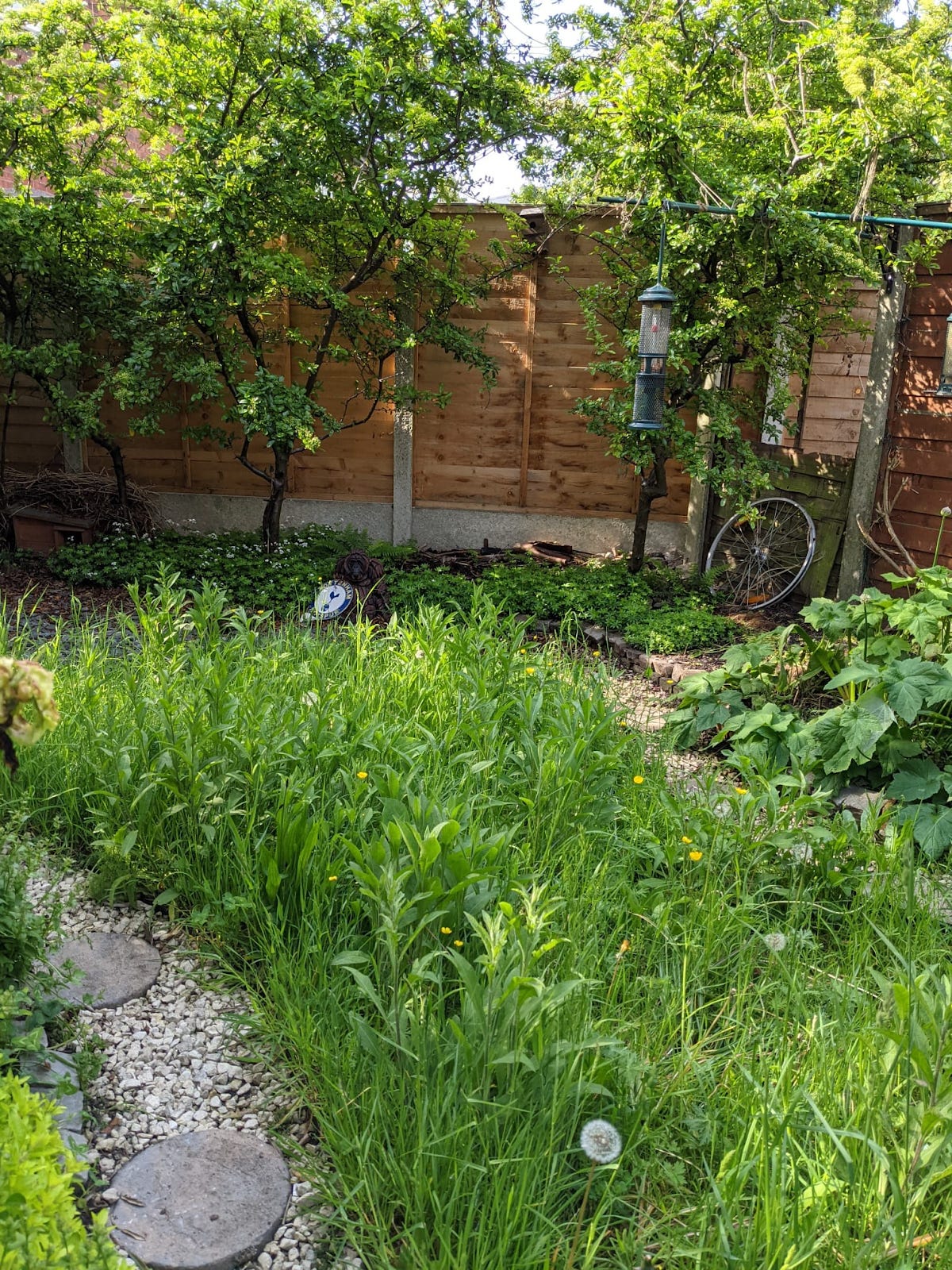The image captures a lush, slightly overgrown backyard scene with verdant grass and tall greenery, giving it a wild, natural feel. Centered in the scene is a curving garden path made of gravel and circular stone pavers, which leads toward a light-colored wooden shed with a silver roof. The shed is surrounded by trees and various plants, with yellow dandelions dotting the ground. A prominent wooden fence, approximately seven to eight feet high, stands in the background, with vertical slats and trees growing against it. Against this fence leans an antique-looking bicycle tire, adding a nostalgic touch. Nearby, a green-topped bird feeder hangs from a pole or post. The overall atmosphere of the daylight outdoor scene is both serene and slightly untamed, with a blend of nature and rustic elements.